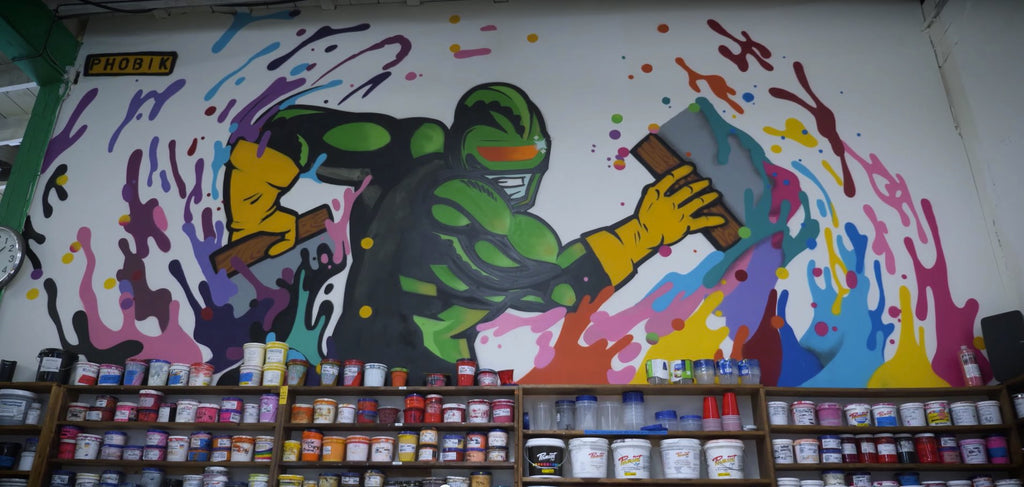The image captures an interior of a paint store, where a colorful and eye-catching graffiti mural dominates the scene. Behind wooden shelves stocked with an array of paint cans and containers, a white wall serves as the canvas for a vibrant artwork. The centerpiece of this mural is a stylized, cartoon-like character reminiscent of a superhero, possibly the Incredible Hulk, rendered in green with pronounced muscles. This character, wearing yellow gloves, a gas mask featuring an orange stripe across the eyes, and blue around the mouth, appears to be in the act of painting. Holding paint scrapers in each hand, he exuberantly spreads a riot of colors—pink, purple, blue, yellow, orange, red, and teal—across the wall in dynamic splatters and streaks. To the left, a distinctive detail includes a yellow box with graffiti lettering that reads "PHOBIK", adding a personal artist's tag to the mural. Further adding to the scene's texture and depth, a clock with a green strap hangs vertically on the left side. The entire composition not only showcases the array of paints available for sale but also creates a unique, engaging visual experience, emphasizing creativity and the vibrant potential of the products.